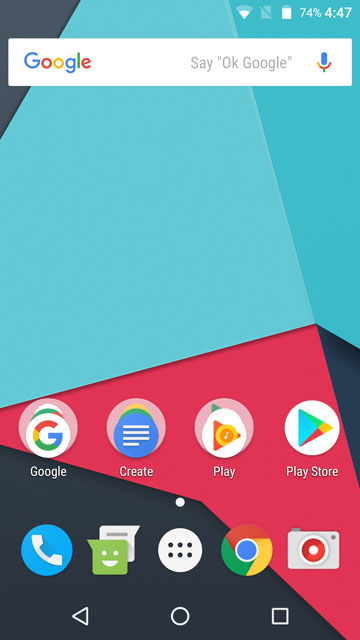The image features a smartphone home screen with a vibrant and visually rich background. The upper half of the background is predominantly a blue-teal color, interspersed with various shapes: a black triangle in the upper left, a smaller black triangular shape on the right, a red triangular shape, and another black four-sided object on the left. 

At the very top of the screen, a status bar displays the Google logo in full color on the left, followed by the prompt "Say 'OK Google.'" Additionally, the status bar shows the battery level at 74%, the time as 4:47, and various other status icons.

On the home screen itself, the interface is divided into rows of app icons. The first row includes:
1. The Google app, represented by the Google 'G' logo within a white circle and labeled "Google."
2. A 'Create' app, featuring a white circle with blue top and white lines, labeled "Create."
3. The 'Play' app, depicted with a red arrow on a yellow circle, labeled "Play."
4. The Google Play Store app, shown as a white circle with a blue, red, and yellow triangle, labeled "Play Store."

The second row displays another set of five icons:
1. A blue circle with a white phone icon.
2. A green square icon with two eyes and a mouth, superimposed on a white square.
3. A white circle displaying six black dots aligned in two rows of three.
4. A blue circle featuring a smaller white circle encircled by red, yellow, and green rings.
5. A gray file icon, distinguished by a white circle encircled by a red ring and a subsequent white ring.

At the bottom of the screen, navigation icons are set against a black background: a left-facing triangle (back button), a circle (home button), and a square (recent apps).

Each element is precisely detailed, contributing to a dynamic and organized smartphone interface.